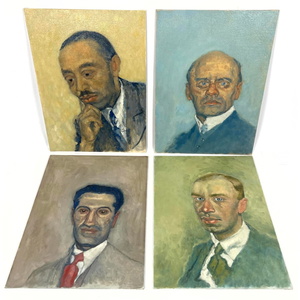The image is a collection of four distinct portraits of men, each placed in its own quadrant with solid-colored backgrounds. In the top left, a dark-skinned man with a receding hairline and tiny black hair follicles, is depicted against a yellow backdrop. He is dressed in a gray suit with a blue tie, resting his right hand thoughtfully on his chin while looking down at a 45-degree angle, showing no emotion.

In the top right quadrant, set against a blue background, there is an older, light-skinned man with a stern expression. He is bald with sparse hair on the sides and wears horn-rimmed glasses. Dressed in a black suit and a white high-collared shirt, he stares straight ahead.

The bottom left quadrant features a dark-skinned man against a brown background. He has short black hair and is dressed in a tan suit, complemented by a white shirt and a red tie. This man also appears emotionless, looking straight ahead.

Lastly, the bottom right quadrant shows a light-skinned man with a slightly red complexion and a five o'clock shadow against a green background. He has receding blonde hair and deep furrows in his brow. He wears an olive green suit with a matching tie and a white shirt, also looking forward without any apparent emotion.